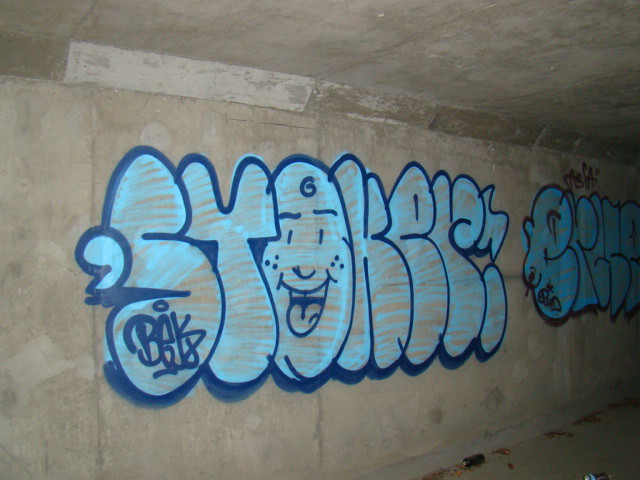The image depicts a gray, stone wall under an overpass or possibly inside a tunnel or subway setting, adorned with elaborate blue graffiti. This graffiti showcases large, bubble-shaped letters with a dark blue outer edge and a lighter blue interior, accented by intentional gaps revealing the stone color. Central to the design is a character face within the letter 'O,' playfully sticking its tongue out. The text appears to start with "S-Y," potentially includes "K-E-R," and features another indistinct word. The artist's signature is visible on the initial 'S,' flanked by small symbols. Additional details in the scene include a can on the floor and the ceiling structure above, indicating an urban environment with sufficient lighting.